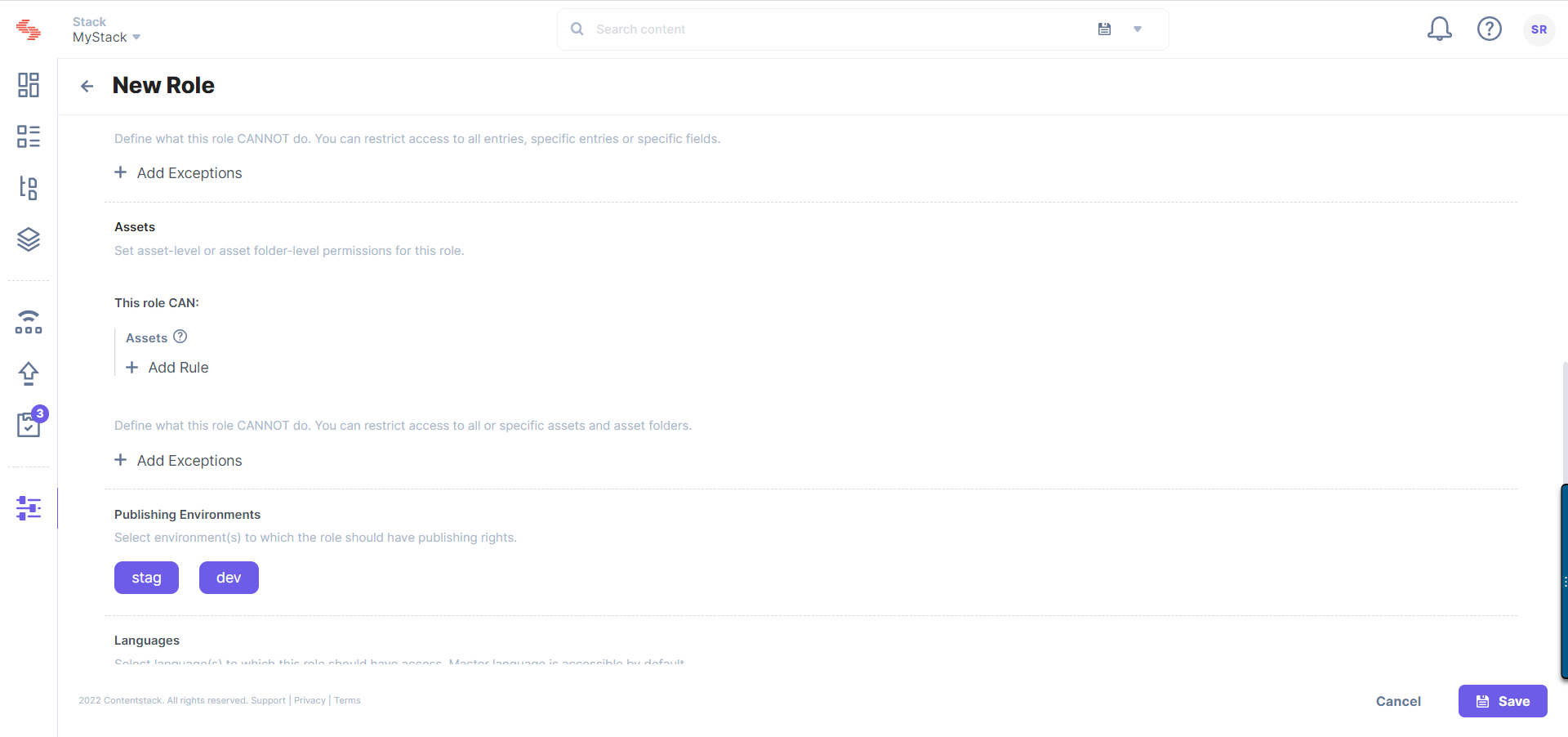The image displays the "MyStack" program, currently on a profile screen. 

In the top right corner, there are three icons: a circle with the initials "SR", a question mark inside a circle, and an alert bell. At the center and top of the page, there's a search box labeled "Search content," which also features a save disk icon. On the far left, there's a logo for "Stack" with a dropdown menu option labeled "MyStack".

Below this header, the section titled "New Role" appears in bold with an arrow pointing to the left. Underneath, the text reads: "Define what this role cannot do. You can restrict access to all entries, specific entries, or specific fields." There is a button labeled "Add Exceptions" with a plus symbol next to it.

The next section is titled "Access Assets." Below it, the text states: "Set access level or access folder level permissions for this role." It continues with: "This role can: Access." There is an "Add Rule" option with a plus symbol adjacent. Further down, it mentions: "Define what this role cannot do. You cannot restrict access to all specific assets and assets folders." Another "Add Exceptions" button with a plus symbol is present.

Following, the section "Publish in Environments" includes the instruction: "Select environments to which the role should have publishing rights." Two purple buttons are available: one labeled "STAG" (S-T-H-E), and the other "DEV" (D-E-V).

The final section pertains to languages, although the text is partially cut off. At the bottom right-hand corner, there are options to "Save" and "Cancel".